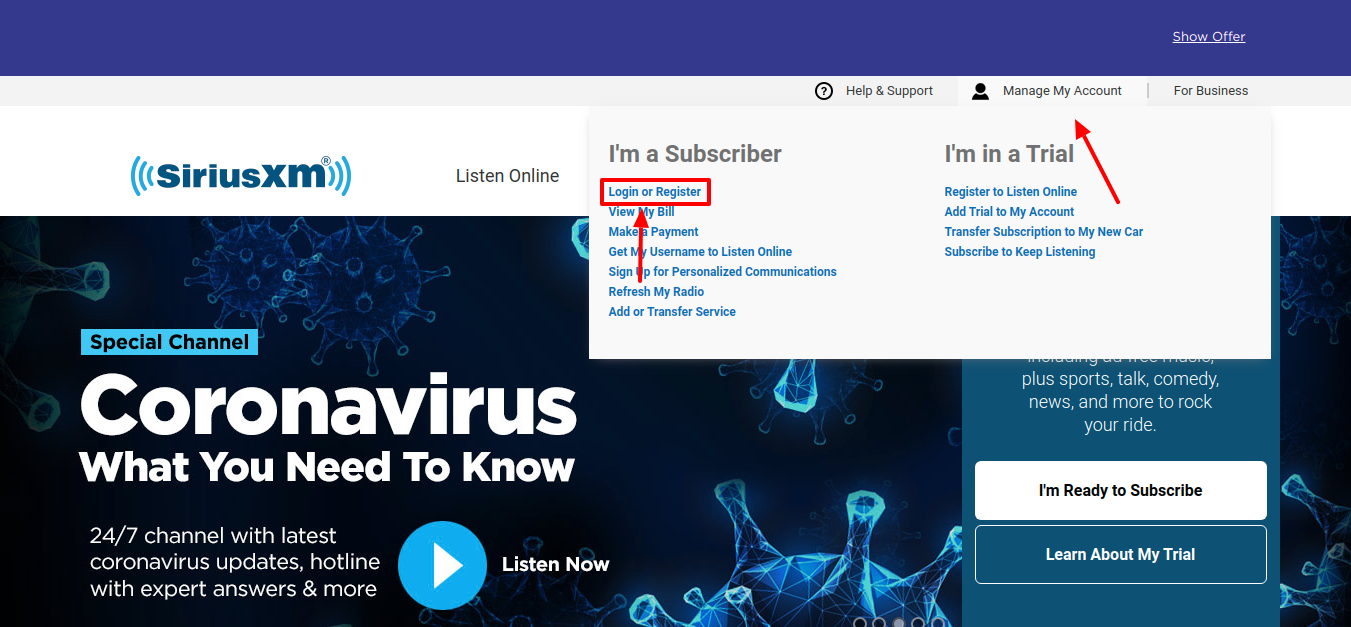The image depicts a webpage from the SiriusXM website that prominently features a COVID-19 advertisement. The webpage has a dark navy blue navigation bar stretching across the top. In the upper right corner of this bar, a prominent white button labeled "Show Offer" is visible. Directly beneath this, a light gray bar spans the width of the page, followed by a white bar below it. 

In the center-left portion of the white bar, the SiriusXM logo is displayed, flanked by stylized blue sound waves. To the right of the logo, a button labeled "Listen Online" is situated. On the right side of the webpage, there is a dropdown menu with options for "I'm a Subscriber" and "I'm in a Trial," indicating user access points.

Visible within this dropdown, both the "Login" and "Register" buttons are highlighted in red, accompanied by red arrows pointing to "Manage My Account." Below these elements, a special channel titled "Coronavirus: What You Need To Know" is featured, suggesting dedicated content related to the pandemic. 

Based on the highlighted "Login" or "Register" button and the "Manage My Account" section, it appears the user might be experiencing an issue related to account access or sign-in status.